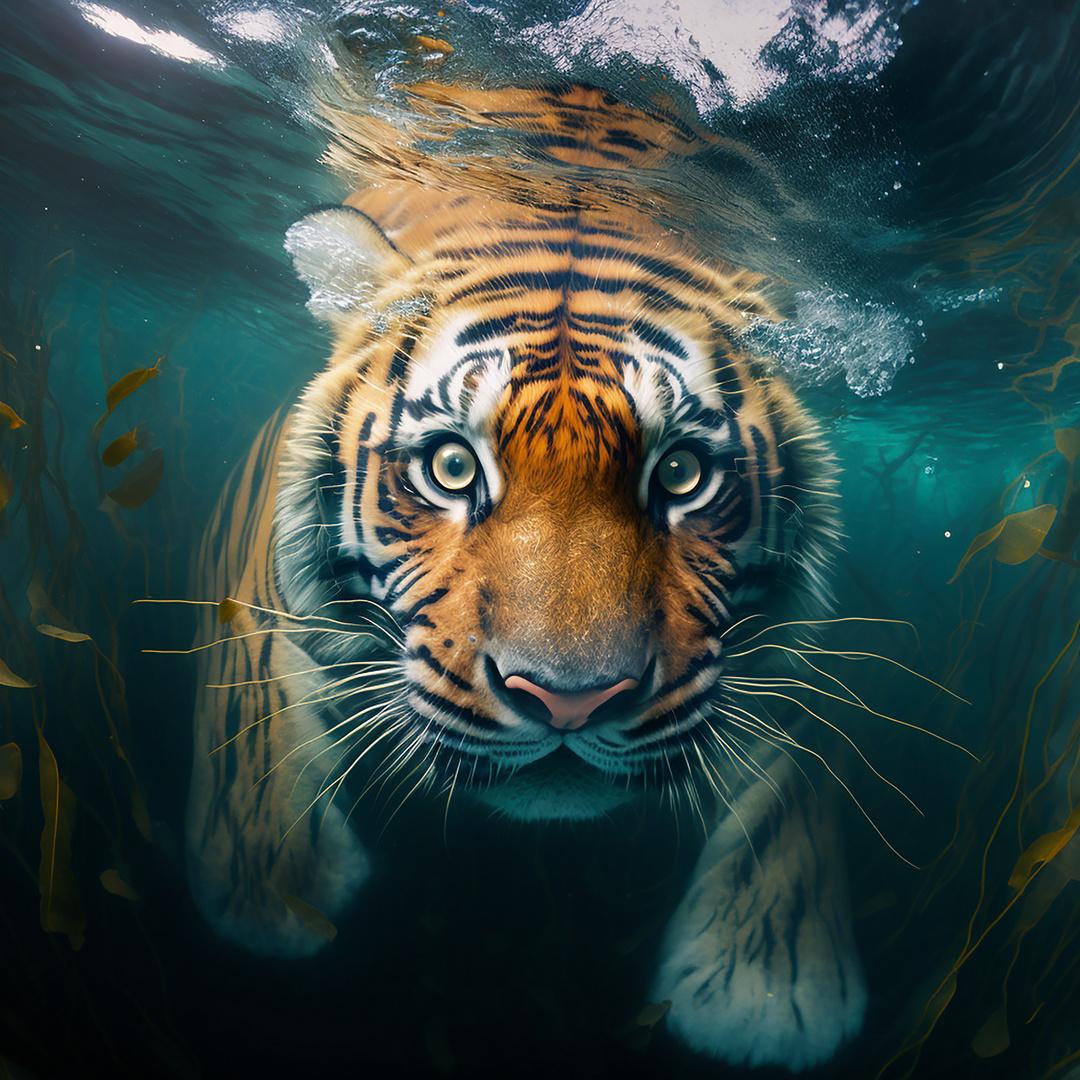In this vividly detailed AI-generated image, an animated tiger with striking, regular black stripes and golden eyes is partially submerged in water, displaying a mixture of realism and digital artistry. The tiger, orange with white ears and a white backdrop, appears to have just leapt into the water. Its wide, expressive eyes give it a slightly surprised look, as if it’s adjusting to the aquatic environment. The tiger's numerous whiskers are prominent as it swims, its paws paddling visibly. Around it, fish swim peacefully, undisturbed. Elements like seaweed are present, adding to the underwater scene's authenticity. The overall clarity and detail suggest that this is more of a digital painting or a heavily edited photo, possibly created by artificial intelligence, capturing an imaginative and captivating moment that would have been nearly impossible and highly dangerous to photograph in the wild.